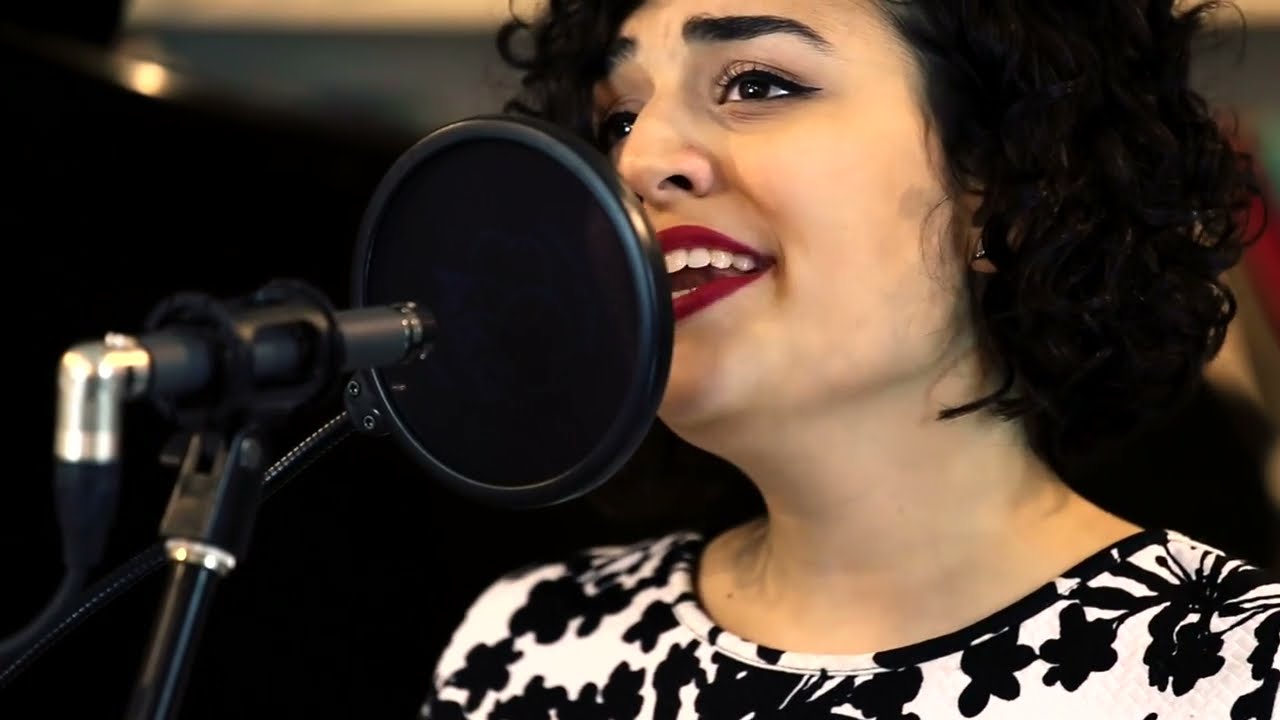In this detailed color photograph, a sophisticated musical ensemble performs live amidst the literary ambiance of a library, characterized by an extensive backdrop of colorful book-filled shelves. Central to the image is a woman with light skin, dark hair, and dark eyes, elegantly dressed in a black and white floral print dress, singing passionately into a microphone. To her left, a young man with brown hair and a beard, dressed in a black suit, white shirt, and tie, is seated, playing a grand piano with a brown interior, on a black bench. On her right stands another gentleman holding a trombone with a poised readiness, his light skin and brown hair visible, attired in a black suit and red tie, and positioned near a microphone stand and sheet music holder. The performers, in their formal dress wear, harmonize in this inviting and cultured library space, surrounded by shelves brimming with books of varied hues including red, black, white, blue, yellow, purple, pink, and gold. The ground beneath them is a warm tan, adding to the cozy and refined atmosphere of this live musical event.